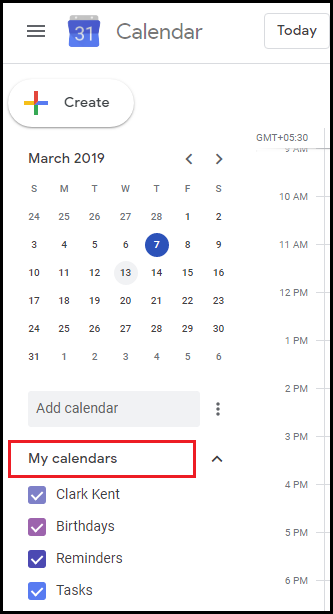The screen capture displays a detailed view of a Google Calendar interface for March 2019. At the very top, three horizontal lines denote a drop-down menu. Adjacent to this menu icon is the number "31" followed by the word "Calendar," indicating the active application. On the top-right corner, there is a text box labeled "Today," along with a Google Plus icon and an oval button for creating new events.

In the main calendar view, navigation arrows allow the user to scroll forward and backward through the months. The days of the week—Sunday, Monday, Tuesday, Wednesday, Thursday, Friday, and Saturday—are listed across the top. Specific attention is drawn to March 7th, which is circled in blue, and March 13th, which is grayed out to signify an event.

At the bottom, there is an option to add a new calendar. The "My Calendars" section is highlighted with a red box around it, indicating it has been selected. Within this section, individual calendars such as Clark Kent, Birthdays, Reminders, and Tasks are displayed with check marks beside each, showing they are active. On the right column, the time zone is specified as GMT+5:30.